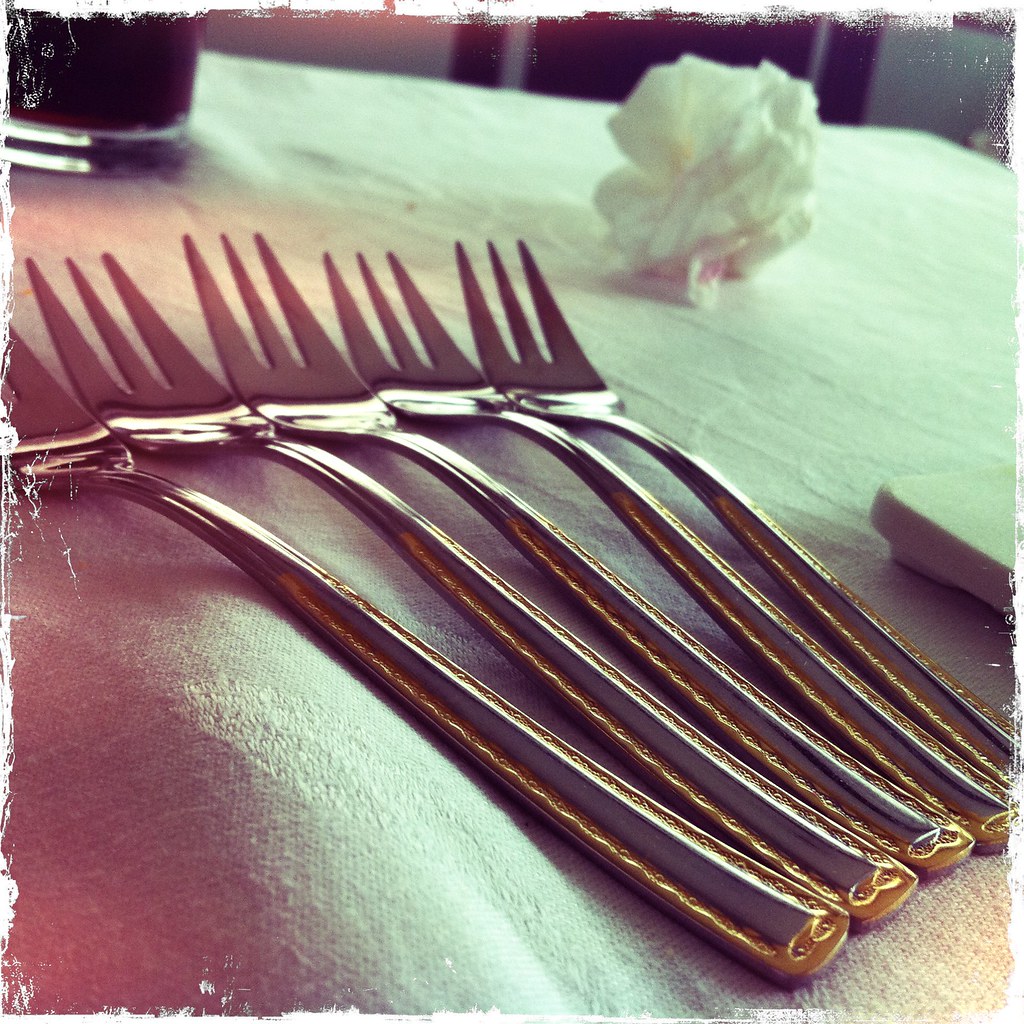The image displays five silver forks, each with three prongs, laid closely together on a white textured tablecloth. The forks feature intricate golden decorations along their handles. Surrounding the forks, the scene includes a crumpled white napkin, the rounded corner of a plate, and in the top left corner, a drinking glass or vase containing a dark liquid. The photograph has an intentional vintage style, with faded, worn edges, resembling an old-time photo effect.